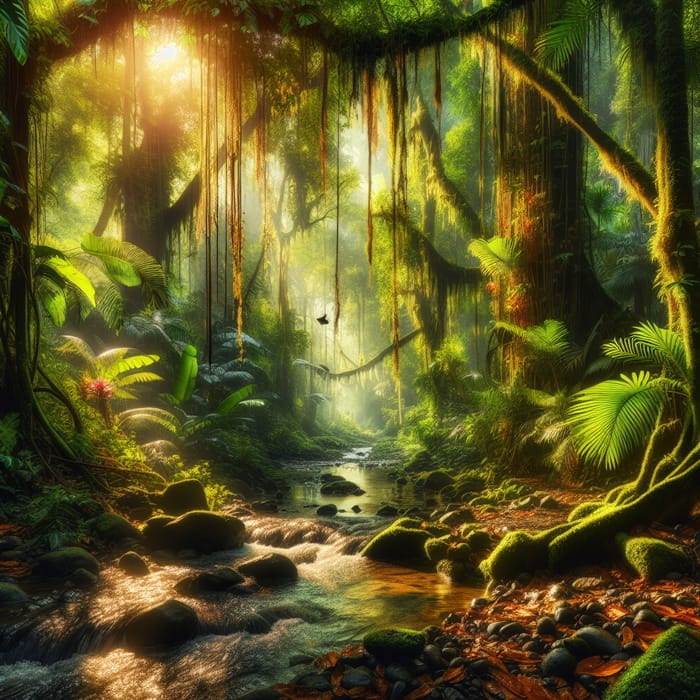This is a detailed and vibrant depiction of a lush jungle or rainforest scene, crafted with a smooth digital animation style, potentially AI-generated or heavily digitally edited. The square image showcases a central stream flowing over rocks, cutting elegantly through the middle. Surrounding the stream are tall trees on both sides, their brown trunks supporting an array of green ferns, bushes, small flowers, and grasses. Vines, some golden, hang down from the branches, adding a touch of whimsy to the scene.

In the upper left corner, a bright, red-hued Sun shines through the trees, casting a dramatic and vibrant yellow glow across the entire image. This brilliant light, which also pours through the branches, creates strong contrasts with deep shadows, especially noticeable on the right side. A large tree trunk with moss and vines occupies the upper right corner, while the bottom right reveals a patch of brown dirt or mud with scattered black rocks. The vivid coloration and the interplay of light and shadow give the forest a shimmering, almost magical appearance.